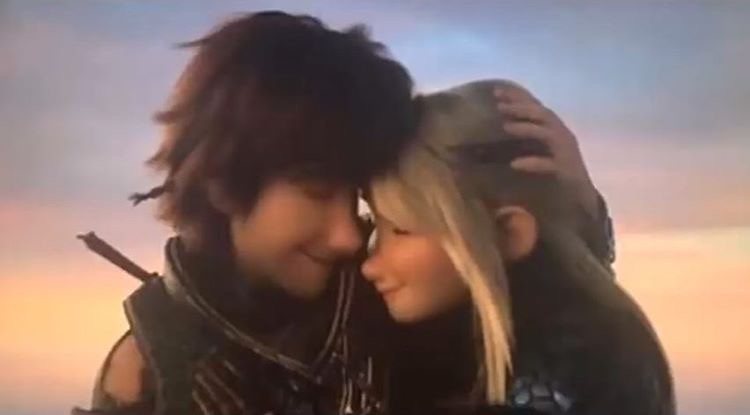This is an illustration depicting two computer-generated characters, a man and a woman, embracing closely with their foreheads touching. The man, positioned on the left, has short brown hair and wears a brown leather protective garb with a sword on his back and a metal breastplate. His left arm is wrapped tenderly around the woman's head, which he gently holds. The woman, on the right, has long blonde hair and a smile that suggests a deep bond between them. She appears to have an outfit with snake-like patterns or stones on her shoulders, hinting at a warrior-like attire similar to the man's. The background features a sky gradient transitioning from blue at the top to shades of red, orange, and yellow towards the bottom, evoking a sense of dawn or dusk. Both characters have their eyes closed, emanating a feeling of serene affection.